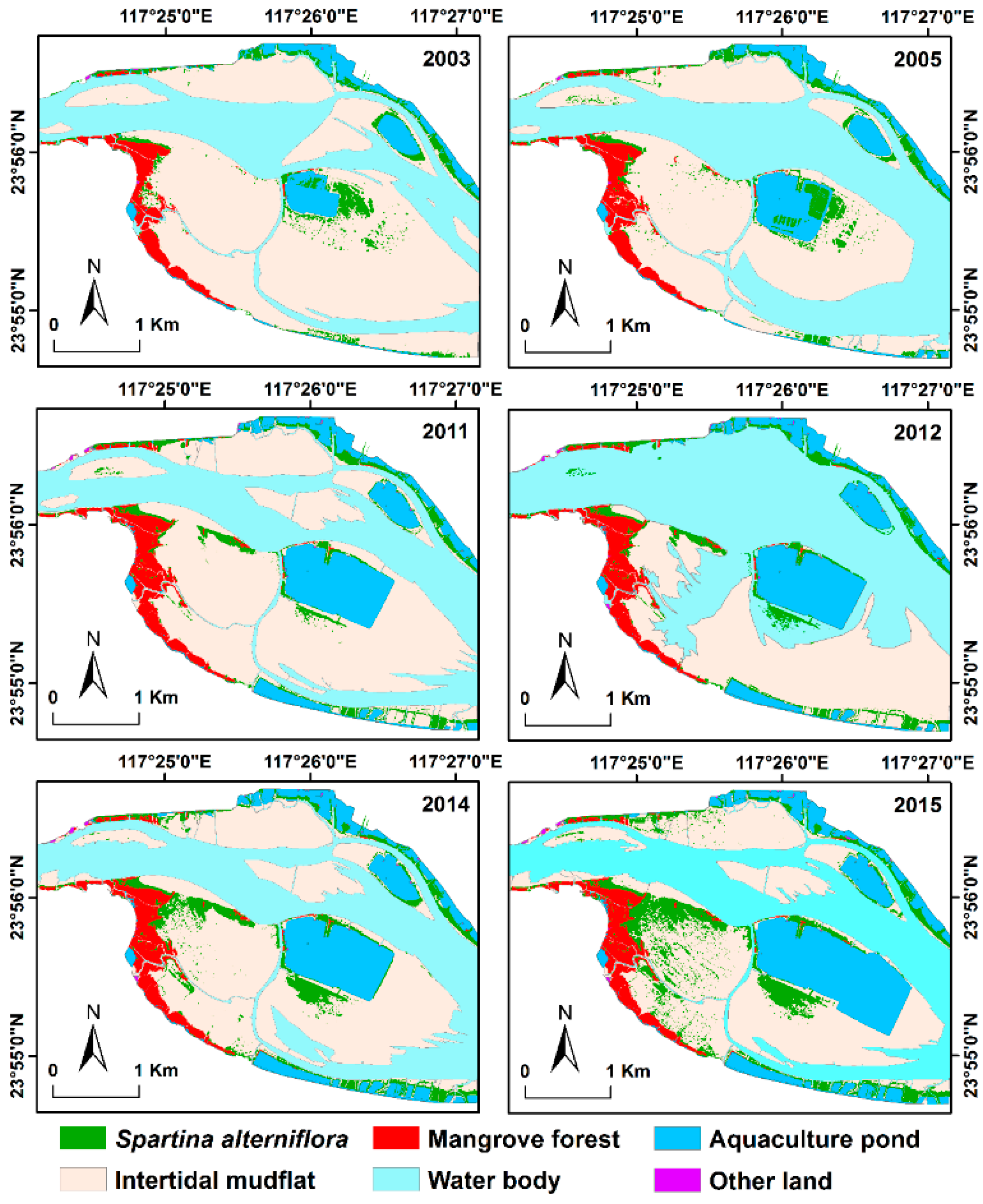The image depicts a detailed, color-coded diagram of a geographic region, presented as six maps aligned in a grid. Each map, set against a white background, represents changes in the landscape of the same area over different years: 2003, 2005, 2011, 2012, 2014, and 2015. The maps are detailed with directional coordinates, showing latitude along the top and longitude on the right. The diagrams are color-coded to indicate various land types, with green representing Spartina Alterniflora, pink for intertidal mudflat, red for mangrove forest, cyan for water bodies, dark blue for aquaculture ponds, and purple for other land. A legend is provided at the bottom, explaining the color codes. This comparison vividly shows the periodic changes in land use and vegetation across the years, highlighting the evolving landscape dynamics in this region.